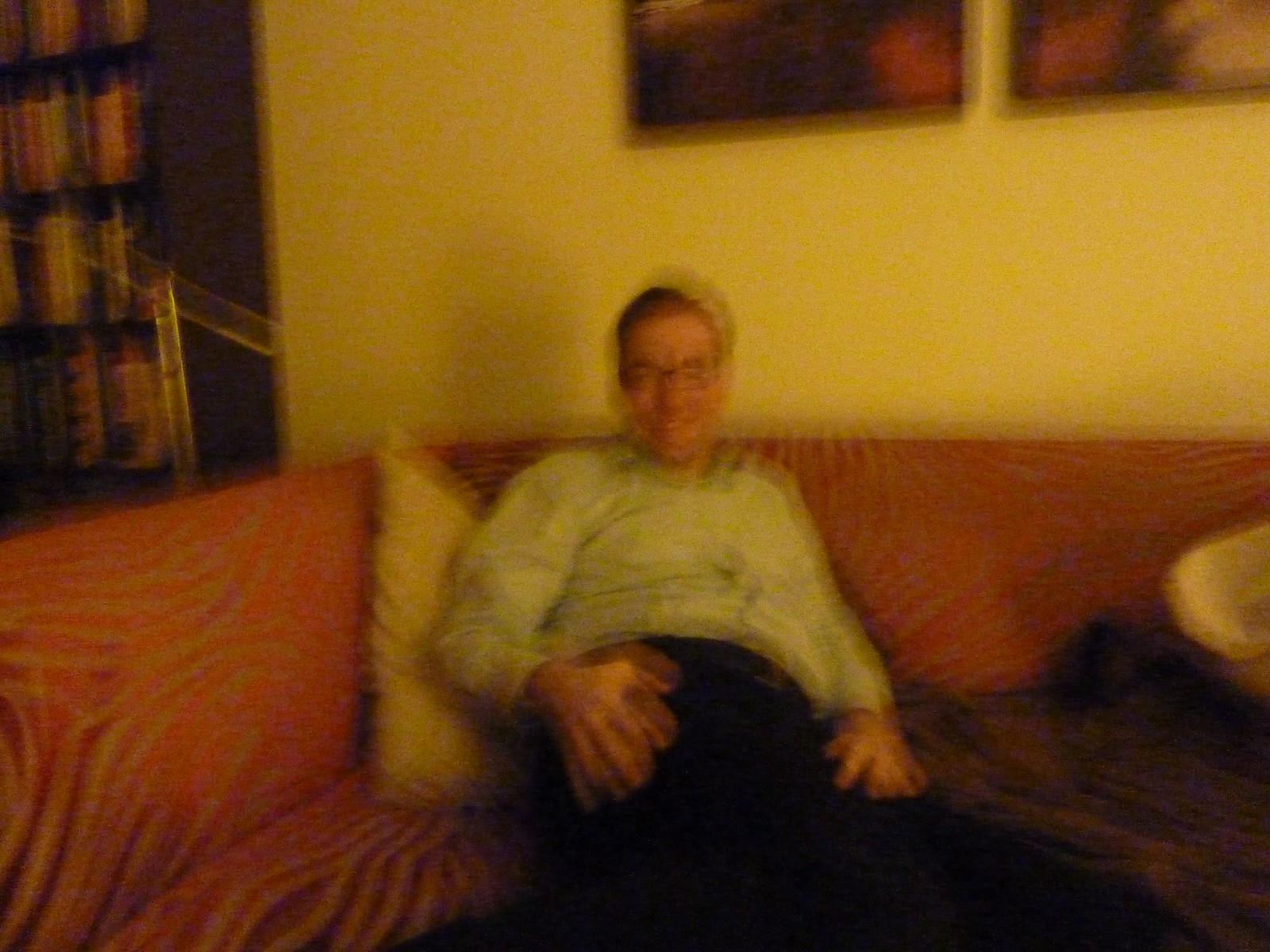In this very blurry photograph, a smiling Caucasian man with short brown hair and glasses is sitting back on a corner couch in what appears to be a living room. The man, dressed in a light-colored or gray long-sleeved button-down shirt and dark or black pants, has his left hand on his upper hip and his right hand on his upper thigh. His head is slightly leaning back, yet he remains easily recognizable. The couch he sits on is red with white or gray stripes and includes an orange sheet and a yellowish pillow behind him. The wall behind the man is yellow, adorned with two paintings in brown frames, though only the bottom halves are visible. To the man's left is a bookcase stacked with rows of books. The lighting in the room has a yellow hue, adding warmth to the scene.